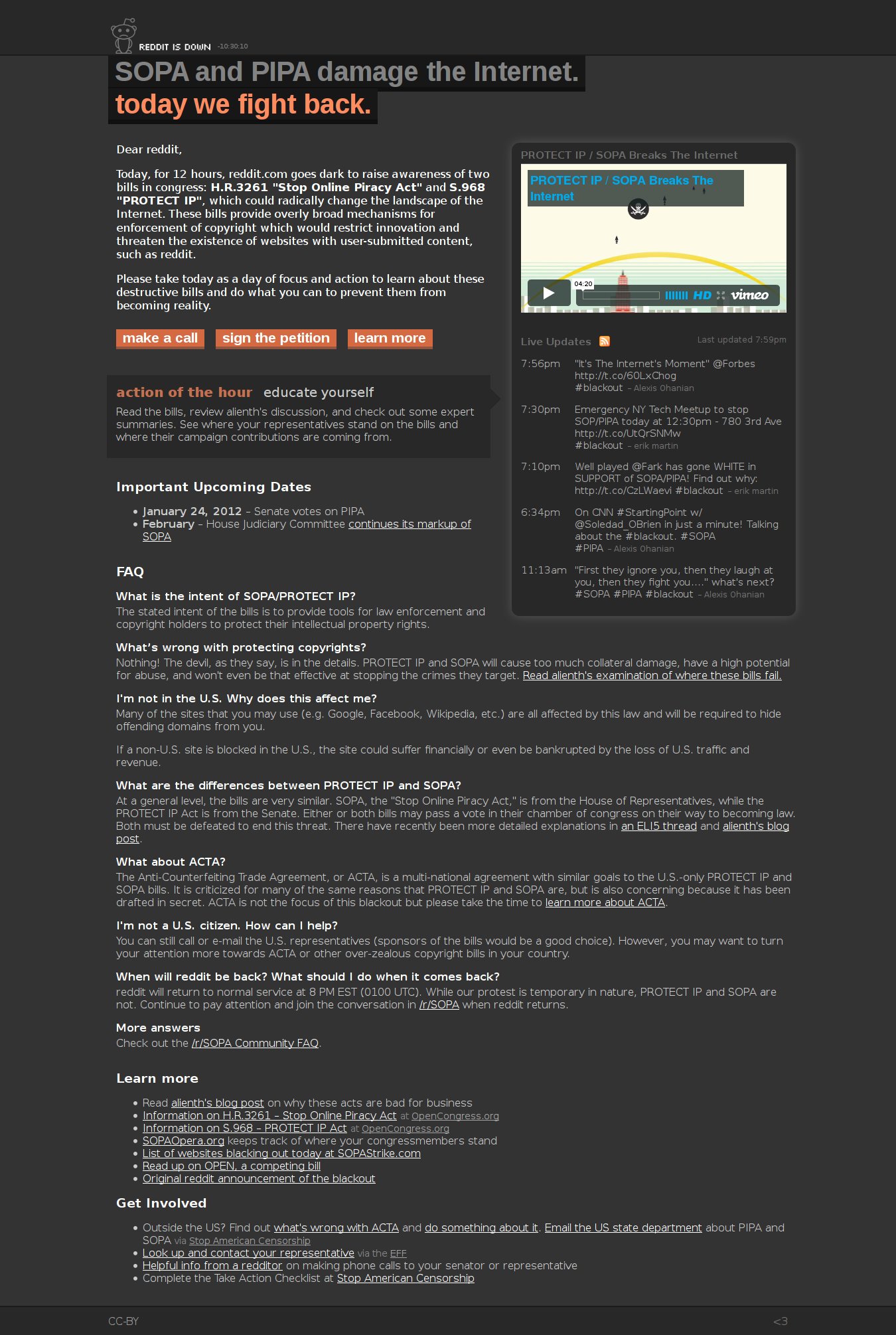**Screenshot of Reddit's Anti-SOPA/PIPA Campaign Page**

The image showcases a detailed screenshot of a page from Reddit advocating against the SOPA and PIPA bills. At the top, a clear and prominent message announces, "Reddit is Down," with a sad-faced Reddit alien icon, signaling the site's temporary blackout.

The headline reads, "SOPA and PIPA Damage the Internet: Today We Fight Back," introducing a long, comprehensive article. The opening paragraph starts with "Dear Reddit," and explains that for 12 hours, Reddit.com is going dark to raise awareness about the detrimental effects of these two Congressional bills.

Beneath the introductory text, there are three conspicuous, orange rectangular buttons:
1. **Make a Call** 
2. **Sign the Petition**
3. **Learn More**

Another section titled "Action of the Hour" appears nearby, encouraging users to educate themselves further about the bills. Important dates are highlighted below this section, with January 24th, 2012 being the first listed, followed by dates in February.

The page continues with an FAQ section featuring about seven or eight popular questions for more clarification. Sections for "Learn More" and "Get Involved" provide additional resources and ways for users to participate in the fight against SOPA/PIPA.

On the top right-hand side of the page, a prominent video box titled "Protect IP/SOPA Breaks the Internet" offers live updates and can be played on Vimeo, providing a dynamic understanding of the issues at hand.